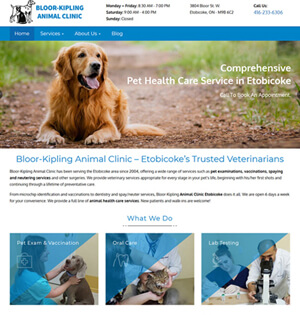Top left features an image of a Dalmatian with text overlay reading "Bloor Kipling Animal Clinic." The caption provides essential contact information, stating the clinic is open Monday, Friday, Saturday, and Sunday, and can be reached at 416-238-6306. Services listed include "Home Services," "Abidas," "Bongs," and "Blue Bar," which points to a Golden Retriever on a dirt road with leaves and grass. The clinic offers "Comprehensive Vet Healthcare Services." A call to book an appointment is encouraged.

Prominently, blue text highlights "Bloor Kipling Animal Clinic," "EW Coke," "Trusted Veterinarians," and mentions surgery supervision and general services. In response to the question, "What do we do?," the text portrays numerous veterinary services provided by the clinic: "Pet Exams," "Vaccinations," and "Oral Care." There's also an illustration of a blue triangle at the top left, while the bottom right shows a dog sitting. The caption further details lab testing, showcasing a cat scratching, lab testing symbols such as a microscope, test tubes, scrubs, and a lab coat. There is a humorous reference to "Donkey Dong" towards the end.